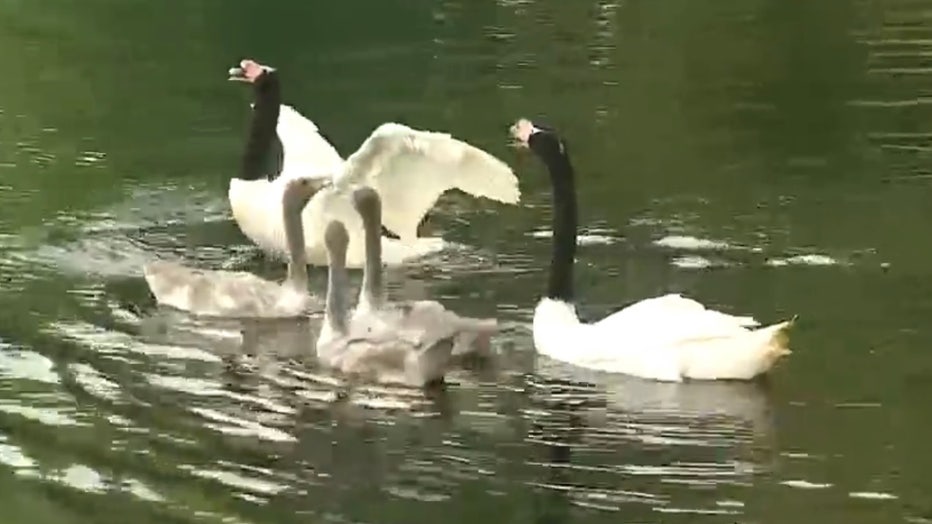This photograph, likely a still taken from a video due to its slightly out-of-focus and low-quality appearance with visible compression artifacts, captures a family of geese in a murky, greenish lake. The image, taken during daytime with soft sunlight creating light reflections on the slightly rippled water, shows two adult geese with striking black necks and pure white bodies, sporting light reddish heads and gray-colored beaks. Alongside them are three juvenile geese, displaying lighter gray bodies with darker gray necks and heads, their beaks also gray. One of the adult geese appears poised to flap its wings, adding a dynamic element to the scene as the family swims together in the tranquil, somewhat murky waters of the lake.